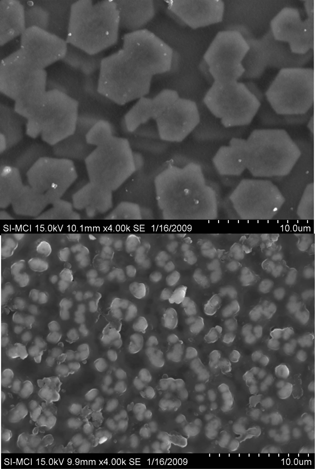The vertically aligned rectangular image displays two grayscale photographs taken through a microscope, possibly a scanning tunneling microscope, capturing different sections of a material's surface. The top image showcases irregular, gray shapes, some resembling stacked octagons, set against a darker gray background. Below this, a black strip contains white text: "SI-MC1 15.0 KV, 10.1 millimeters x 4.00 K SE, 1/16/2009," with "10 microns" on the right side. The bottom image is similar but features a collection of smaller, gray clusters with a few white pieces. This section also has a black strip at the bottom with text nearly identical to the top, except "9.9 millimeters" replaces "10.1 millimeters," retaining the same date and "10 microns" detail. The images together provide a detailed, magnified view of the material, with the top likely being a closer view due to the larger appearance of the objects.